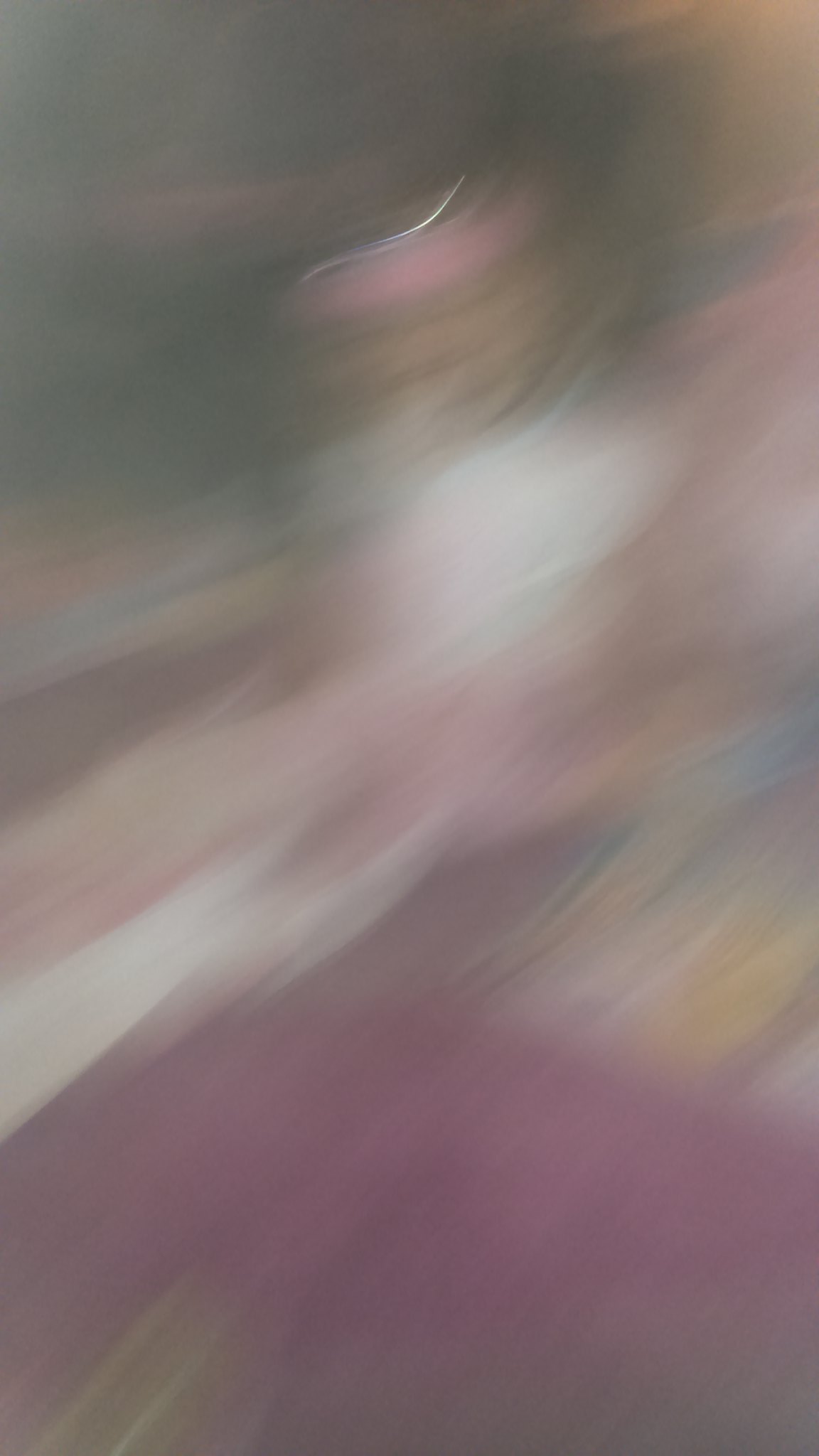This out-of-focus, rectangular image presents a dreamlike blend of colors and shapes that suggest an abstract painting. Dominated by a gray and pink theme, with what appears to be a face faintly discernible beneath the layers of color, the composition transitions into patches of white, possibly indicating an outfit or shirt. The image becomes increasingly saturated toward the bottom, evolving into rich shades of pink, purple, and a distinctive green streak emerging from the lower left corner. The upper region features a mix of yellow, white, and blue hues that meld into gray, interspersed with swirls of purple. The top is predominantly gray with touches of pink. Amidst these overlapping colors, brown, blue, and tan elements also surface, contributing to the impression of a person within a painting or a series of abstract forms, as viewed through a veil of blurriness.